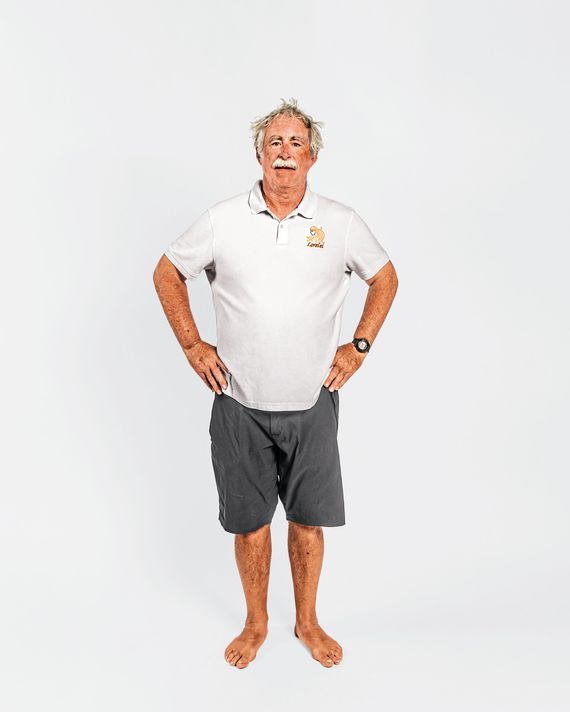An older gentleman, possibly in his mid-60s to early 70s, is standing barefoot against a stark white background, which gives the impression of a studio setting. He is wearing a short-sleeved white polo shirt with a small, unreadable logo where a pocket might be. His gray khaki shorts reach his knees, and he sports a black digital watch on his right wrist. His light-complected skin features red splotches on his arms and legs. The man has scraggly, sandpaper-gray hair, bushy gray eyebrows, and a thick white mustache, giving him a slightly disheveled appearance, as if he has just woken up. He stands with his hands on his waist, looking at the camera with an expression of curiosity or confusion.